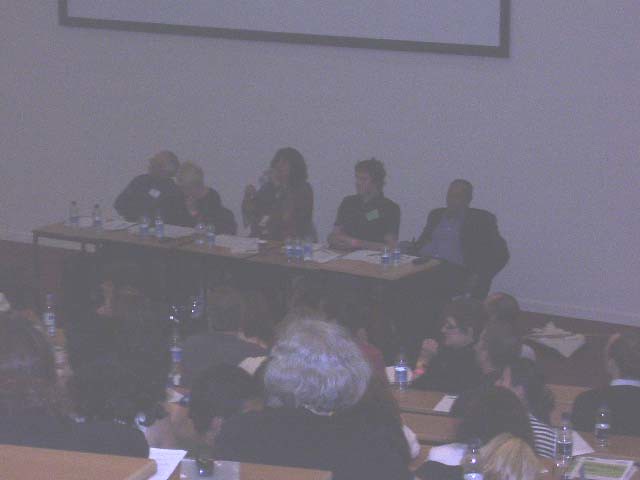The photograph depicts a faded and blurry indoor setting of what appears to be a college classroom with stadium-style seating. At the front, there is a white wall featuring a large whiteboard, above which hangs a movie screen. Five individuals are seated at an elongated desk cluttered with papers and water bottles wrapped in blue labels, suggesting they were distributed beforehand. The individuals—a mix of men and women, one with notably gray hair—are looking outward toward an indistinct audience. The audience is seated in a tiered arrangement that tapers downward, reminiscent of auditorium seating. Attendees, seen mostly from the back, also have water bottles, papers, and books laid out before them. One person is discernible to the side, wearing glasses. The backdrop of the scene includes glimpses of additional brown wooden desks. The overall color tone of the photograph is grayish, adding to its blurred and indistinct quality.